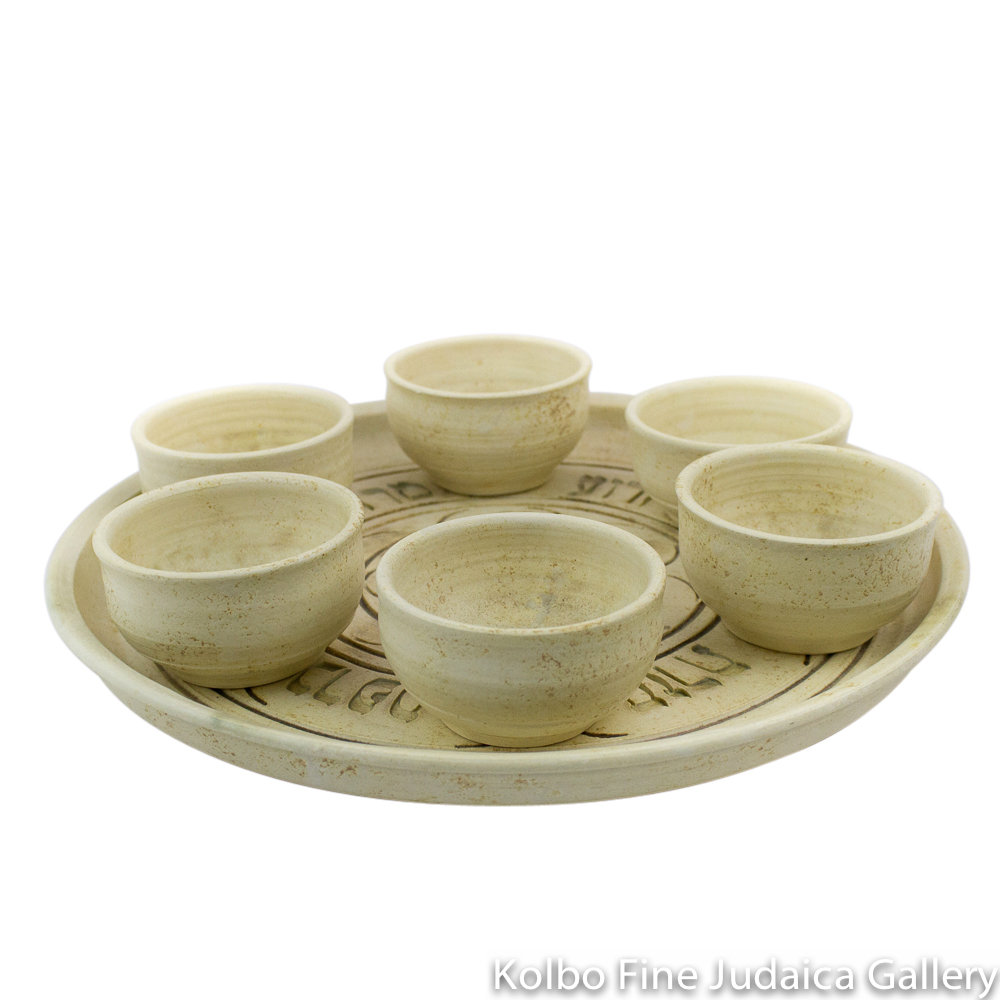The photograph features a stoneware set against a white background, prominently displaying a round beige and speckled brown tray with etched Hebrew letters partially obscured by six simplified stoneware cups. The arrangement on the tray is circular, with each cup varying slightly in height but unified in their roughly painted off-white, tan, and brown hues. The platter, which bears the inscription "Kolbo Fine Judaica Gallery" at its base, showcases a pattern of large circles mostly hidden by the cups that take up nearly the entire surface of the tray.